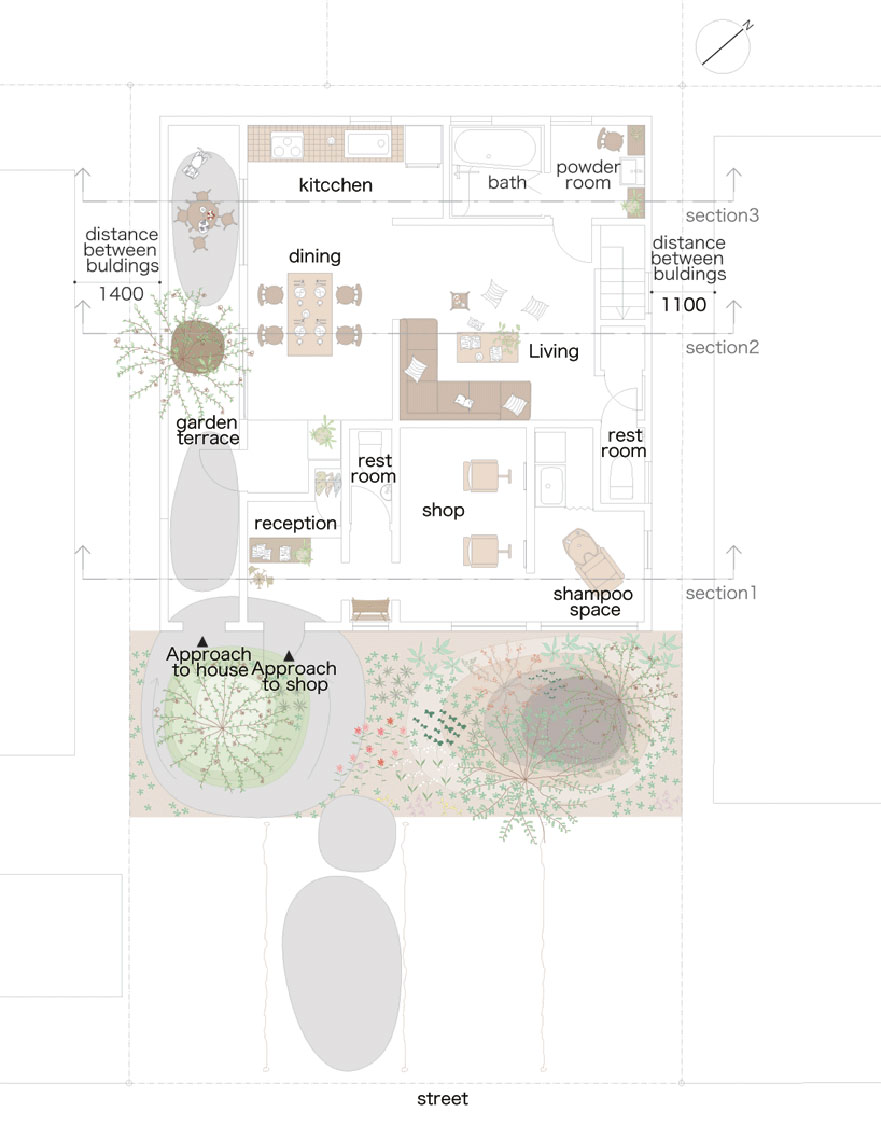This blueprint depicts a mixed-use building that includes both residential and commercial spaces. At the bottom of the blueprint, the street is labeled. Above the street, there are labeled circles denoting the 'approach to house' and 'approach to shop,' indicating separate entrances for the residential and business areas. The layout includes detailed sections labeled such as kitchen (misspelled as K-I-T-C-C-H-E-N), bath, powder room, living area, dining area, and restroom. The blueprint also shows the garden terrace and various outdoor elements like plants and trees in front of the home. Distances between buildings are noted, with one of them measuring 1,400. Specific areas like 'shampoo space' and multiple sections (one, two, and three) are included. From the description, this building could function as a space where one can operate a business, possibly a shop with a reception area, while also residing within it, evidenced by the living and dining areas.